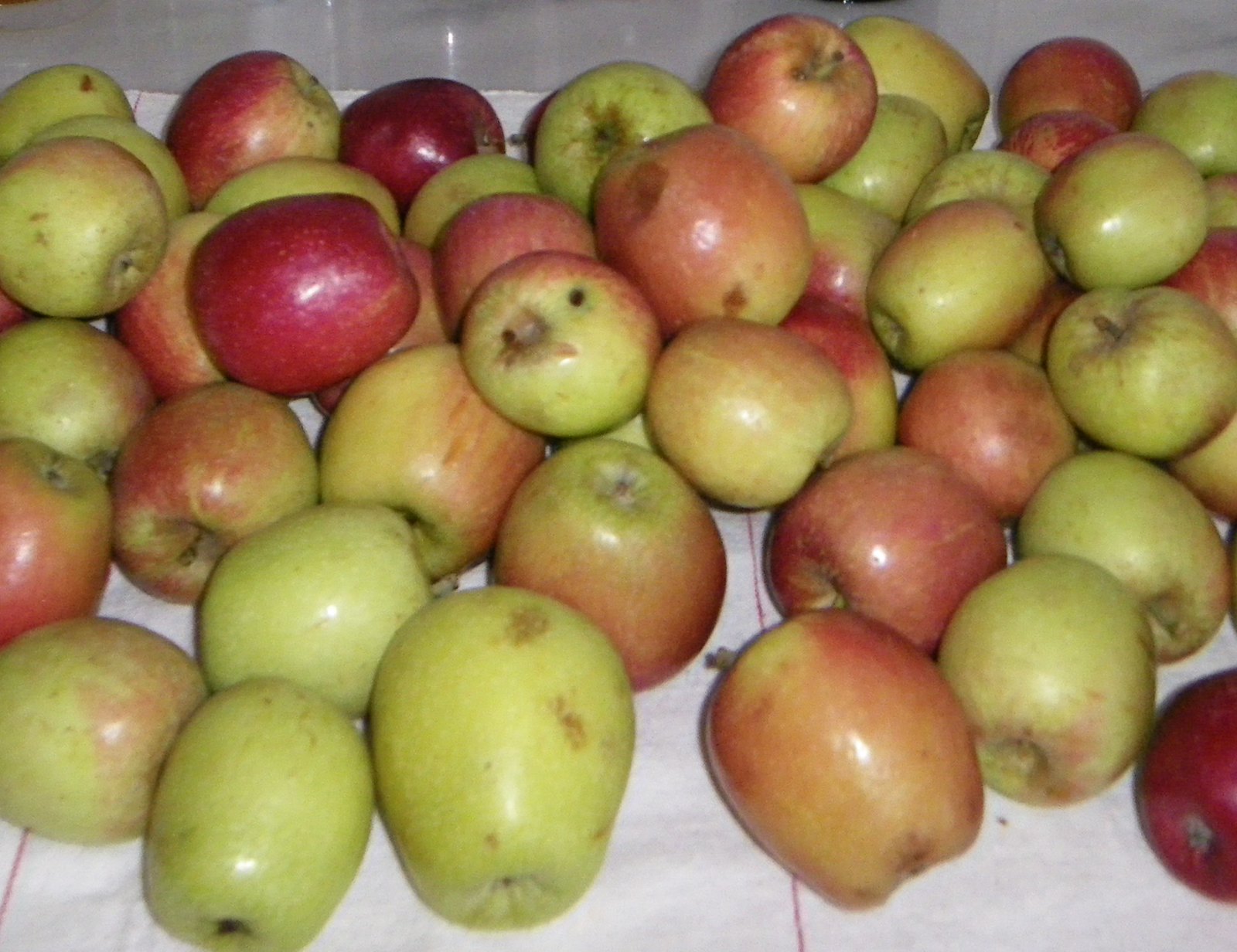This is a detailed indoor photograph, taken with flash, capturing a pile of apples likely freshly picked from a garden tree. The apples display a variety of colors, predominantly green and red, with many showcasing a blend of both hues. They rest on a white, marble-effect tiled surface with narrow bands of red cement in between the tiles, and a grey-tiled wall is partially visible at the top of the image. The apples vary in size and shape, with some being more round and traditionally apple-shaped, while others are larger and slightly more misshapen, resembling a pear. Despite being in various states of freshness, there are noticeable bruises, insect damage, and other blemishes. Some apples still have their stems attached. The image conveys a sense of rustic abundance despite the imperfections.